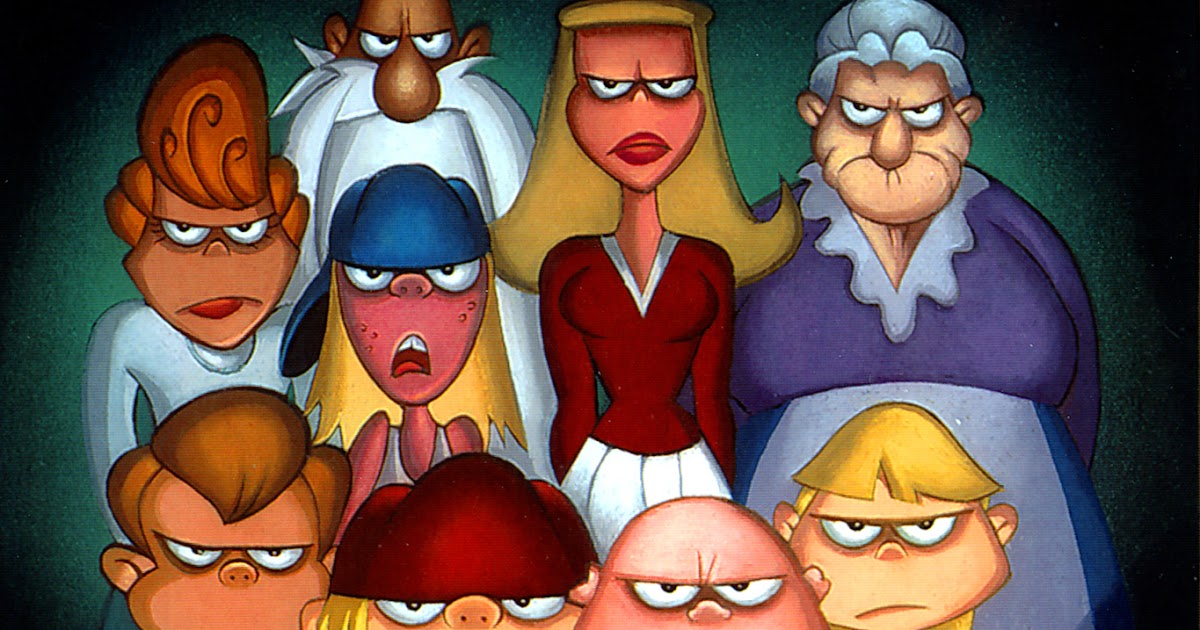A vibrant and humorous cartoon poster features a diverse group of nine characters, each rendered in a casual and fun drawing style. Every figure sports an unusual half-moon-shaped, flowering eye pattern that, combined with their furrowed brows and wide eyes, creates a distinctly angry and astonished expression. The back row includes an elderly woman with a light blue apron and shower cap, a blonde-haired woman in a burgundy top and white skirt, and an elderly man with a white beard and prominent nose. In the middle row, a red-haired boy sticks out his tongue while a girl with blonde hair and an upside-down baseball cap bares her teeth. At the bottom, only the faces of four children are visible: one with a piggy nose and brown mohawk, another with a burgundy cap and tiny, beady eyes, a bald child with a wrinkled forehead, and a blonde boy frowning under a cap. The background transitions from forest green to black, with a blend of color schemes including reds, blues, oranges, and browns adding to the lively scene.